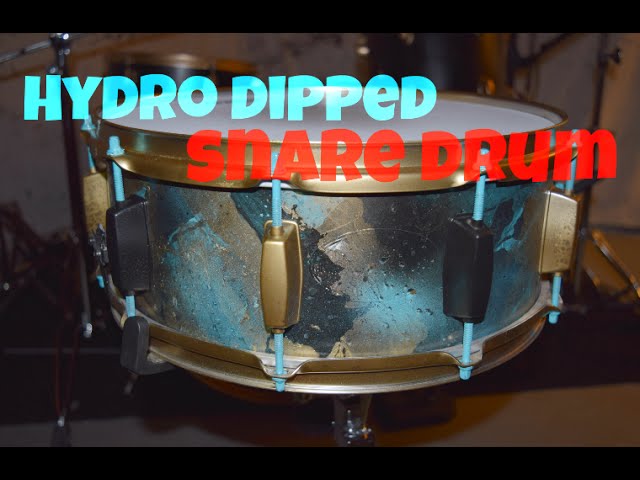The image features a vintage brass or bronze snare drum prominently labeled "Hydro-Dipped Snare Drum" in contrasting text colors, with "Hydro-Dipped" displayed in an aqua blue and "Snare Drum" in red. This unique drum showcases an artistic design on its body, resembling a marble texture with effects of water drops and waves in varying shades of blue and gold, giving it a hydro-dipped look. The snare drum has light blue drum bolts and shiny golden rims, adding to its distinctive appearance. It sits on a metallic silver drum stand, and is part of a larger drum set, as hinted by the presence of other musical equipment, including cymbals with silver stands featuring black legs, blurred in the background. The setup appears to be placed on a wooden bench, enhancing its vintage charm, and the image might have been used as a thumbnail for a YouTube video or an eBay listing due to its cropped format and detailed focus.